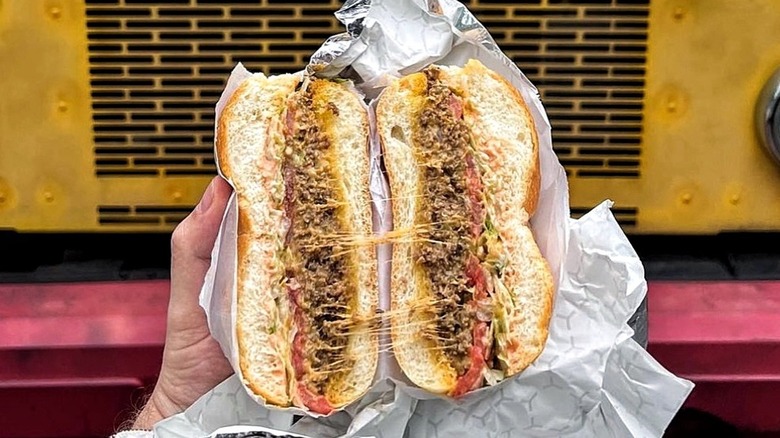A close-up image of a large, foil-wrapped sandwich cut in half, showcasing its contents. The sandwich, likely a chopped cheese or a cheesesteak, is being held by a person with short fingernails, fair skin, and hairy arms, using both hands. Stringy, melted cheese stretches between the two halves of the sandwich, connecting them. The sandwich features pink elements, likely tomatoes or peppers, and is packed with cooked brown meat, some green vegetables, possibly green peppers, and yellow elements such as mustard. It is enveloped in a white sandwich paper with a dashed-line honeycomb pattern inside the foil. In the background, the lower section of the photo is pink, while the upper section features a yellow metal grill, resembling the front of a bus or truck. Part of a silver circle can also be seen on the right side of the image, adding to the mechanical, industrial feel of the backdrop.